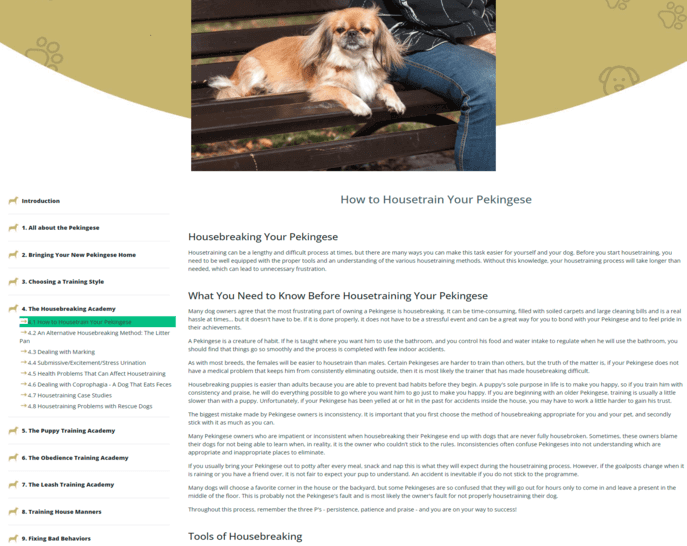The screenshot displays a webpage dedicated to guiding new pet owners through the process of house training their dogs. The left side of the webpage features a vertical navigation menu resembling a table of contents. This menu includes sections such as "Introduction," "All About the Pecking Geese," "Bringing Your New Pecking Geese Home," "Choosing a Training Style," "The Housebreaking Academy," "The Puppy Training Academy," and "The Obedience Training Academy," among others.

The central portion of the page is focused on the "Housebreaking Your Pecking Geese" section, offering detailed advice on how to successfully house train your dog. The text emphasizes the importance of being well-prepared with the right tools and knowledge about various house training methods to streamline the process. Without proper preparation, the house training could be more prolonged and challenging.

The content is presented against a simple background with black text over numerous paragraphs, elaborating on the necessary steps and techniques for effective house training. 

At the top of the page, there is a picture showcasing a dog sitting beside its owner on a brown bench, adding a personal touch to the content. The webpage also features a light brown circular design element adorned with hand-drawn doggy footprints and the outline of a dog, contributing a creative and playful aesthetic to the overall layout.